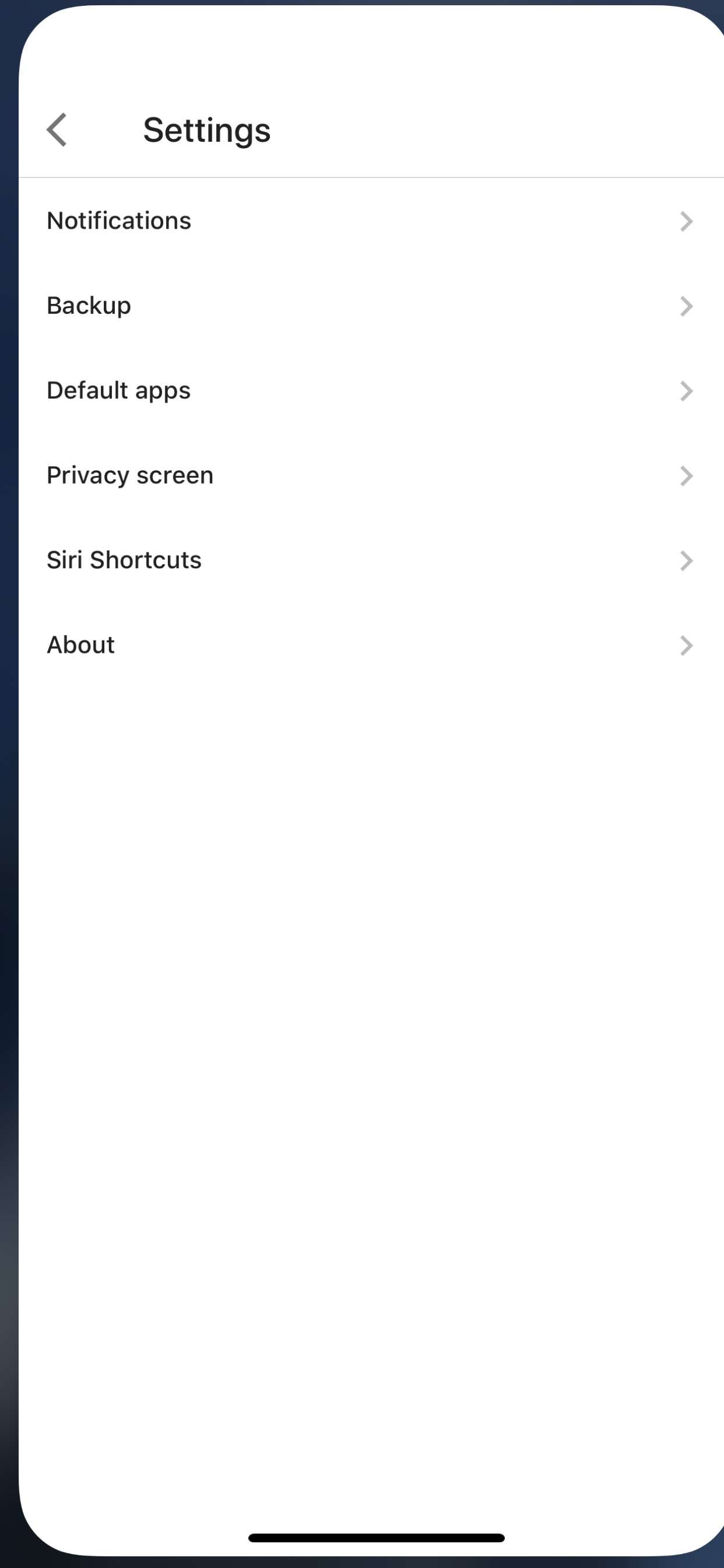Vertical image displaying the settings menu of a smart device. The image features a black border on the left side, which is slightly thicker at the bottom, and a thinner black border at the top. The right side has no border, and the rest of the background is white, likely from the computer screen.

In the upper left-hand corner, there is an arrow pointing to the left, next to the word "Settings" in black text. Below this, a thin gray line separates the header from the menu options. The menu options listed in black text, each accompanied by a clickable arrow, are as follows: Notifications, Backup, Default Apps, Privacy Screens, Siri Shortcuts, and About.